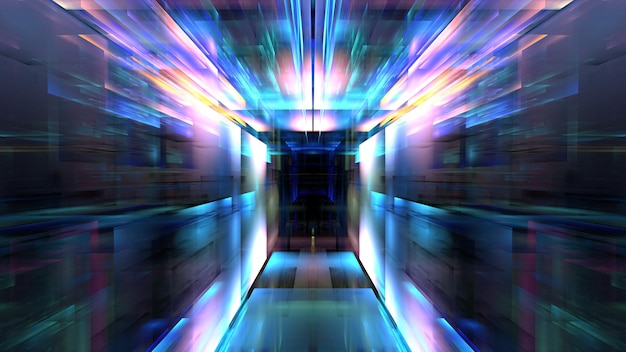The image is a highly detailed, computer-generated rendering of a futuristic, glass-walled hallway illuminated by a vibrant array of neon lights. The narrow passage is lined with translucent walls and a ceiling that reflect and refract light in an array of colors including shades of pink, bright white, light blue, turquoise, mauve, yellow, green, purple, and orange. Neon bars run down both sides of the hallway, creating an ethereal glow that seems to capture reflections of objects not visible within the space. The ceiling's neon effects blend seamlessly with the walls, contributing to the illusion of being inside a prism. The floor is predominantly turquoise and blue, with a striking patch of pink at its center, adding to the hallway's otherworldly aesthetic. At the far end, a dark square opening, tinged with brown or tan at its base, suggests an exit leading to a darker space beyond. The overall effect is one of motion and futuristic ambience, enhanced by the blurred light smears that create a sense of dynamic movement and transform the hallway into a mesmerizing, almost surreal environment.